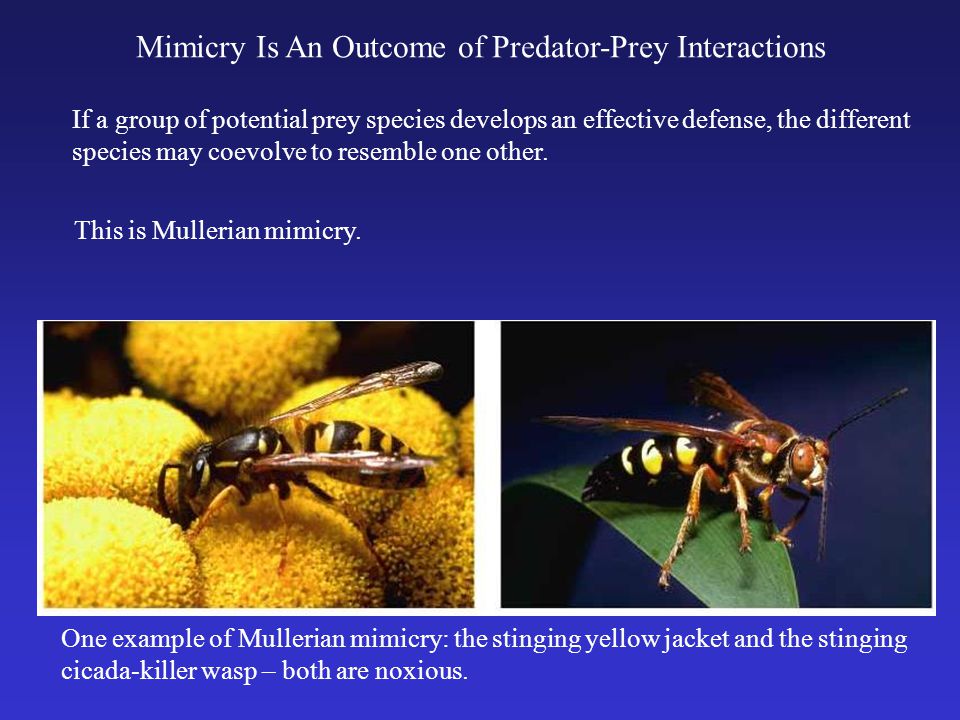The image features a blue background with an informational text about mimicry in predator-prey interactions. At the top, white text explains that "Mimicry is an outcome of predator-prey interactions. If a group of potential prey species develops an effective defense, different species may co-evolve to resemble one another. This is Malarian mimicry." Below this text, there are two photos: the left one shows a stinging yellowjacket, identifiable by its mostly black body with yellow stripes on its abdomen, yellow legs, and long, thin translucent wings. It is pictured on yellow spheres. The right image depicts a stinging cicada-killer wasp with a black, orange, and yellow body, seated on a green leaf. The wasp has thin brown wings, big brown eyes, and black antennae. Additional text at the bottom states, "One example of Malarian mimicry is the stinging yellowjacket and the stinging cicada-killer wasp. Both are noxious." The insects demonstrate how different species can co-evolve to resemble one another, providing an effective defense mechanism in nature.